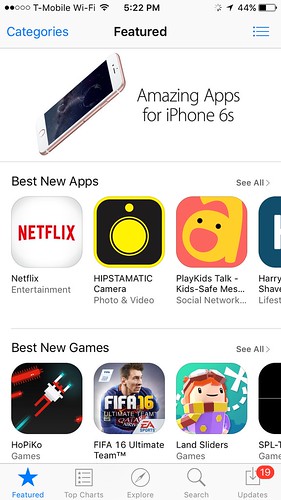The image displays a smartphone interface with various app icons and features. Key details include:

- Network indicators: Two signal dots, Holo's three-dot symbol, T-Mobile, and full Wi-Fi signal.
- Time and status: 5:22 PM, location services active, battery at 44%.
- Interface elements: Categories menu, app size feature, and a hamburger menu.

**Device Description:**
- A black smartphone with white edges.

**Highlighted Apps and Features:**
1. **Netflix**: Entertainment category with a prominent icon.
2. **Hipstamatic**: A camera and photo/video editing app, characterized by a black square icon with white edges, red and yellow center accents.
3. **Messages and Social Apps**: Icons to facilitate communication.
4. **Games**: Notable mentions include:
    - FIFA 16: Ultimate Team, marked with colors red, white, and blue.
    - Landsliders: A game featuring green elements and a character with goggles and a scar.
    - A game titled "Pilla Dash" featuring a blue star icon.

**App Store Sections:**
- Feature section with a "Top Charts" and "Explore" option.
- An update icon depicting a square with a downward arrow.
- Highlighted notifications and offers, including a red banner at the top denoting the number 19.

**Special Mentions:**
- Texas-themed apps for iPhone 6s praised for their quality, specifically mentioning T-Mobile's excellence.
- Reference to the T-Mobile CEO and new games with a focus on vibrant colors such as red, white, and blue.

This detailed caption provides a comprehensive overview of the smartphone's interface, highlighting its network indicators, apps, and key features.